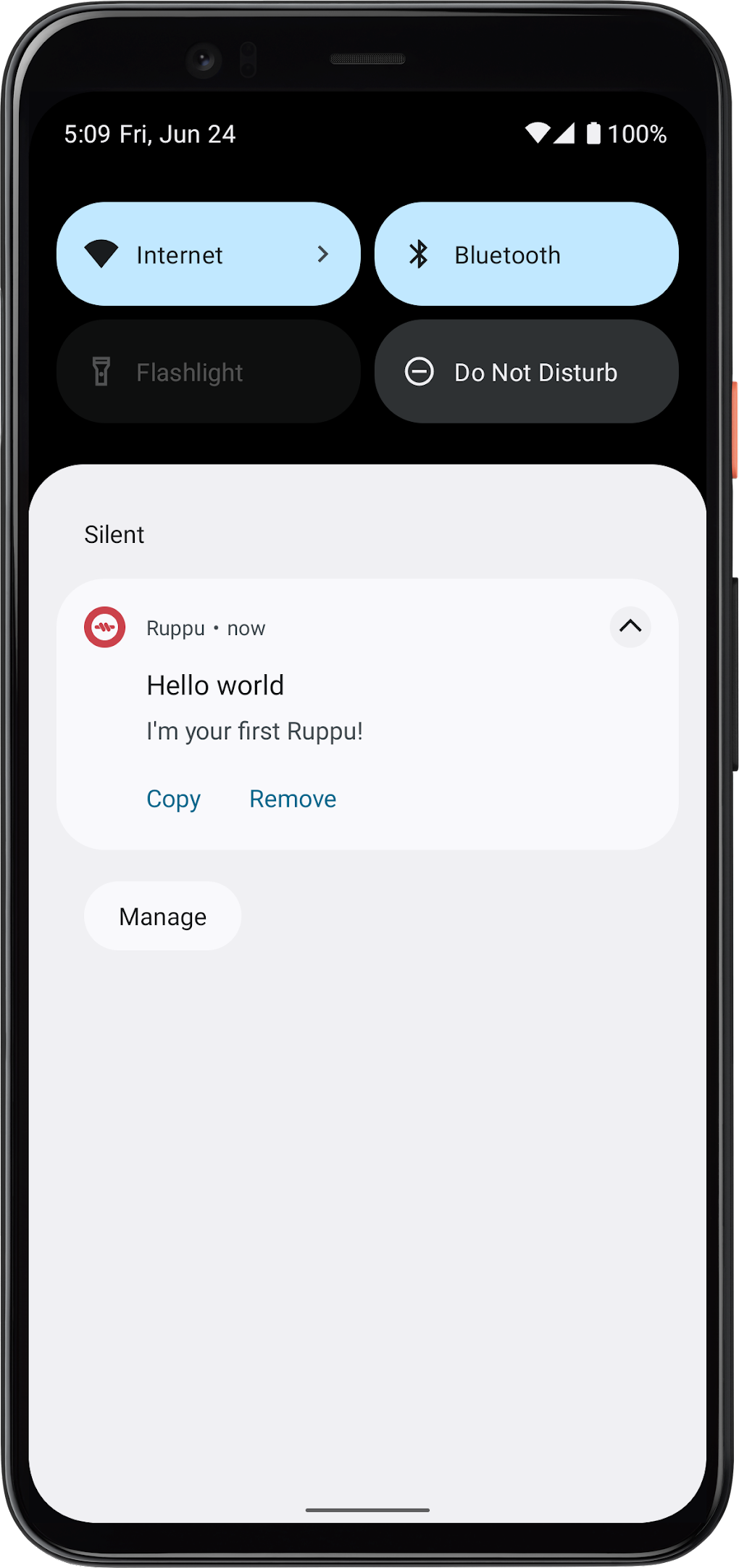A screenshot of a black-outlined smartphone is displayed, showcasing a meticulously detailed phone interface. The upper portion of the phone screen has a black background. The top-left corner shows the time "5:09" in white, followed by "FRI, Jun 24". The phone’s battery, Wi-Fi, and reception indicators all show 100%, with the battery icon also in white due to full charge.

Prominently visible are two side-by-side light blue ovals: one labeled "Internet" in black text, and the other "Bluetooth." Beneath the "Bluetooth" oval, there is a dark gray oval with the text "Do Not Disturb" in white. Near this section is a black oval, blending into the background, with the word "Flashlight" in gray.

Additionally, a gray notification pop-up is visible. In the upper-left corner of this pop-up, the word "Silent" is inscribed in black. Within the notification area is a lighter gray box featuring the text "RUPPU now". Below it, a message reads, "Hello world, I'm your first RUPPU!" followed by an exclamation mark. Options to "Copy" and "Remove" are presented in blue. Further down, another oval is visible with the name "Manish" in black text and a capital "M."